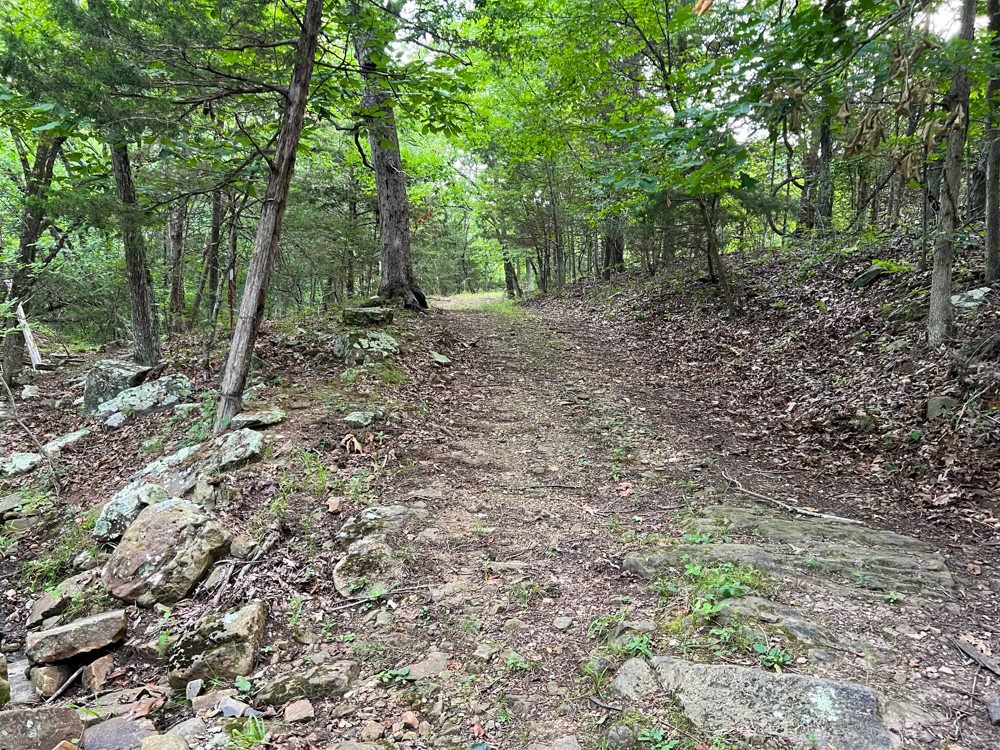The image depicts a rocky path through a forest, taken from the perspective of standing at the trail's edge. The trail, appearing wider in the foreground and narrowing into the distance, is covered with dirt, crushed leaves, and scattered debris from the forest floor. It is mostly shade in the foreground, but a patch of light filters through the trees in the distance, revealing the sunlit road ahead. On both sides, the forest is dense with trees brimming with green leaves. To the left, a notable tilted tree trunk leans back, adding a sense of natural chaos to the scene. The left side also has more rocks compared to the right, where there's a small, raised area resembling a gentle hill. The ground is littered with dead leaves and twigs, with sparse grass and tiny shrubs peeking through. The forest is relatively well-lit, suggesting it's not overly dense, and you can see numerous trees and shrubs, especially concentrated towards the upper parts of the image.